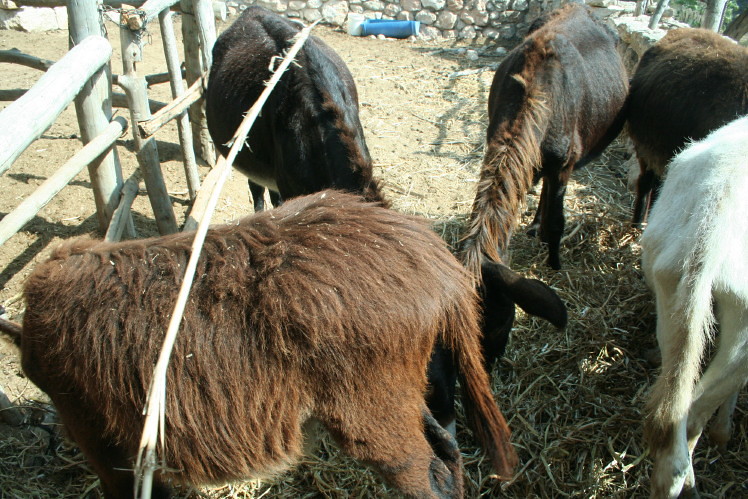This photograph captures a charming outdoor scene featuring barnyard animals within an enclosed area. The background showcases a rock wall constructed from an array of brown and white stones. The ground in the foreground is covered in dirt with scattered hay. To the left, there's a wooden wall that includes a gate secured by a chain, alongside what appears to be a metal enclosure with a pattern of horizontal and vertical lines.

In the foreground, several animals are visible. There is a dark brown animal with long hair, its head turned away, suggesting it's possibly a cow rather than a horse. Near it stands a larger brown animal with short hair, its neck bent down as if grazing, which looks like it could be a horse. Another animal, also dark brown and shaggy, appears to be grazing next to the larger one.

Additionally, you can partially see the backs of two more animals, one brown and one white, indicating they could be cows or horses. To the back and right, there is a black and brown animal, and another white one towards the right edge of the frame. The overall setting is rustic and serene, capturing the harmonious presence of these barnyard creatures.